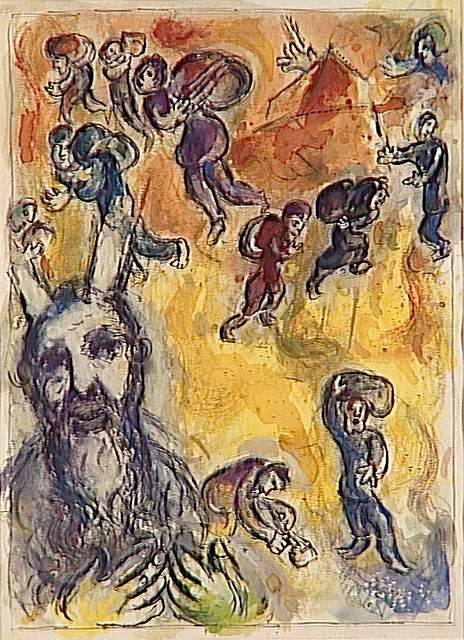This painting, rendered in a style reminiscent of watercolor, presents a somewhat blurry and impressionistic scene dominated by warm hues. The background features a gradient of oranges and yellows, where the orange is more concentrated at the top, gradually blending into yellow towards the bottom. Distinct splotches suggest the application of water to create a flowing, blended effect. 

The composition centers on a large figure in the bottom left corner, an old man with a long beard and a small smile, holding his hands up near his chest. Interestingly, beams of light seem to emanate from his head. His figure, portrayed from the chest up, stands out as the most prominent element in the scene.

Surrounding the bearded figure are approximately ten individuals engaged in various activities. These smaller figures are scattered throughout the image, dressed in an array of blues, maroons, and greens. Many of them appear to be carrying sacks on their backs or bending down to handle objects. One figure in the bottom right notably faces the viewer, holding something on his head and pointing outward.

In the upper right part of the image, there is a structure with a pointed roof, possibly a pyramid, which appears to be orange and engulfed in flames. This adds a dramatic element to the otherwise serene blend of colors. The overall effect is one of dynamic movement and urgency, with a rich tapestry of colors that shift from red and orange at the top, to green and blue at the bottom, encapsulating a vibrant yet distressing scene.